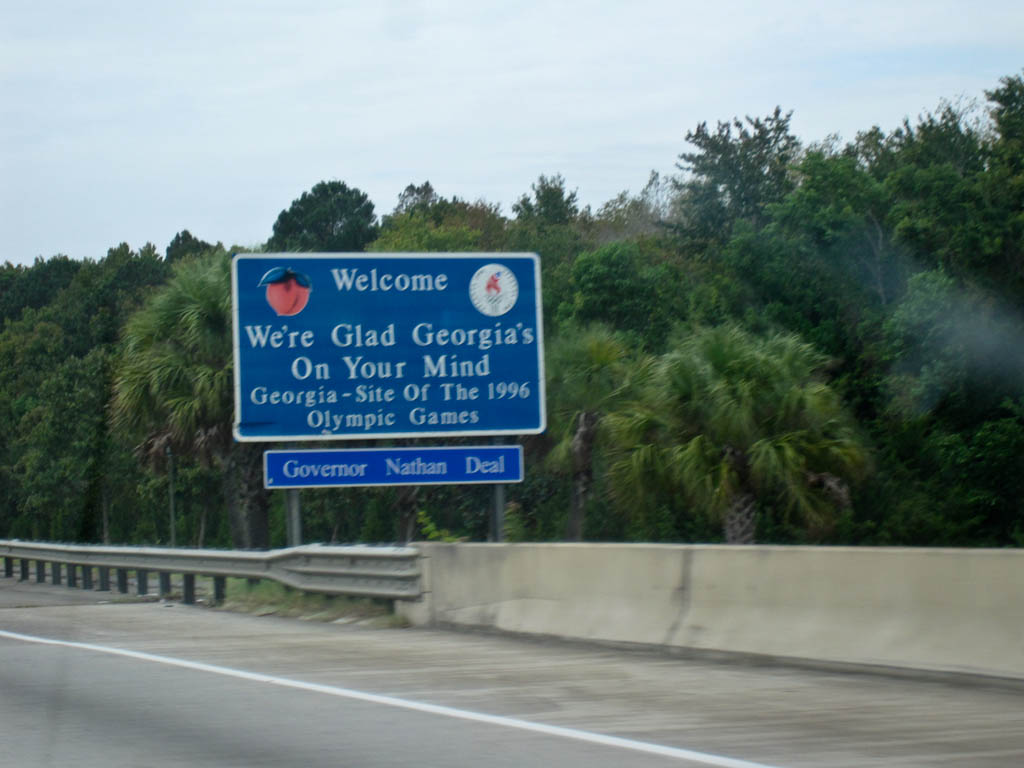In this horizontal outdoor photograph, the viewer's perspective appears to be from a car traveling on a freeway or a merge lane. Prominently featured is a large blue sign on the roadside, welcoming travelers with the message: "Welcome, we're glad Georgia's on your mind." The sign also highlights Georgia as the site of the 1996 Olympic Games and mentions Governor Nathan Deal. The text on the sign is white against the blue background. To the left of the text, there is an illustration of a peach, symbolizing Georgia, and there is an unspecified logo on the right side of the sign that is not fully visible. Surrounding the sign, one can see concrete barriers along the freeway, which are marked by a white line. The scene is framed by abundant greenery, with numerous trees lining the side of the road, reinforcing the outdoor setting of the image.